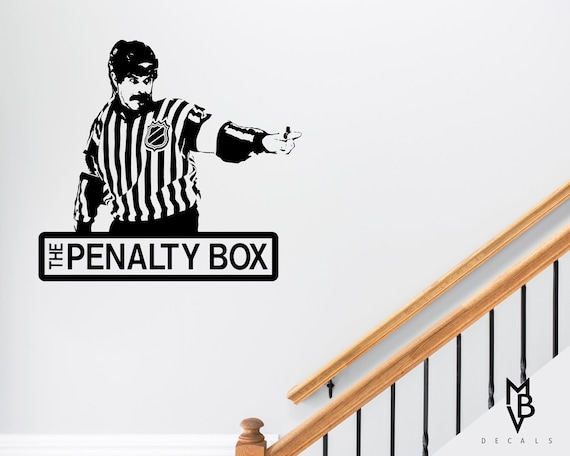This advertising photograph showcases a striking black-and-white wall decal from MBV Decals, known for their sports-themed designs. The image features a blank white wall beside a residential staircase with a light to medium brown banister on one side, accented with black lines, and a banister supported by a newel post and balusters on the other side. The focal point is a large decal depicting an NHL referee wearing a helmet and a vertically striped jersey, complete with the NHL shield logo. The referee, equipped with a whistle in his mouth, points assertively, capturing the intensity of the moment. Below the decal, the caption reads "The Penalty Box," adding context and drama to the scene. In the bottom right corner of the photograph, the MBV logo—forming an artistic arrow with the letters M, B, and V—reinforces the brand's product line, indicating that these sports decals can enhance any flat surface, providing a dynamic and sporty touch to home interiors.